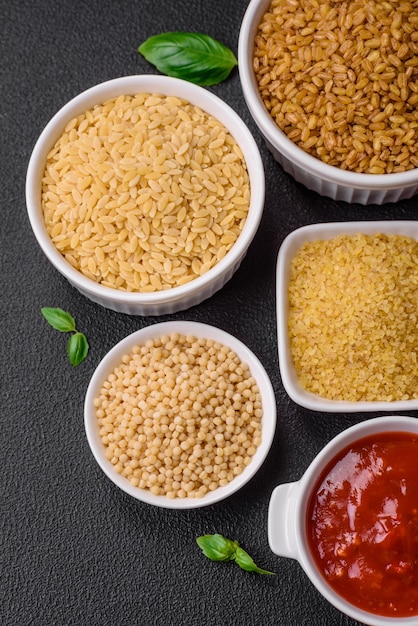The full-color, horizontally rectangular photograph features a professionally staged artistic composition set against a textured blue surface, which may be a table or countertop. Three green leaves are artistically placed: one at the bottom center, one at the top center, and one at the center left. The image includes five white bowls, each rectangular or oval in shape. Three of the bowls are aligned along the right side, while two more are situated towards the center. In the lower right corner, there is a bowl containing ketchup or possibly cocktail sauce. The center-right bowl appears to contain rice, and the other bowls are filled with various grains such as couscous, smaller yellowish grains, and brown rice. The bowls differ in size, with the largest one slightly off-screen in the upper right featuring brown rice. The meticulous placement of the leaves and the varied textures and colors of the grains contribute to the photograph's visually appealing and detailed arrangement.